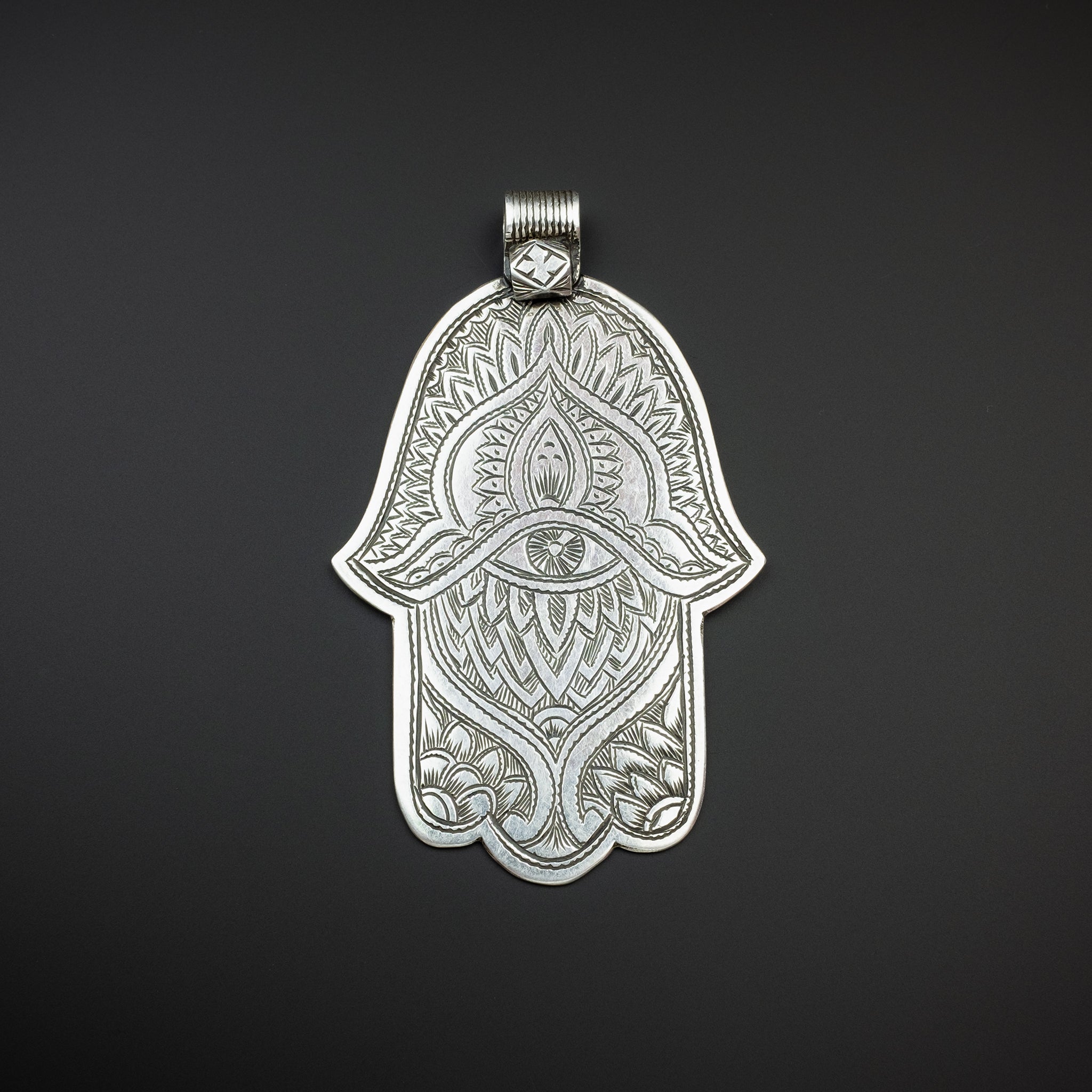The image depicts a detailed, silver Hamsa pendant set against a black background. At the top of the pendant, there is a small loop with a diamond-shaped design, intended for attaching a necklace chain. The pendant itself, reminiscent of a stylized hand, has a distinctive eye in the middle, surrounded by intricate, etched floral and feather-like patterns. These engravings create a three-layered effect, with the feather shapes angling downwards and upwards, almost giving it a mandala-like intricacy. The entire design has a polished, nickel finish with a rope-like edging around the interior. The artistry in the pendant hints at Indian cultural influences, making it both a protective symbol and a piece of ornate jewelry.